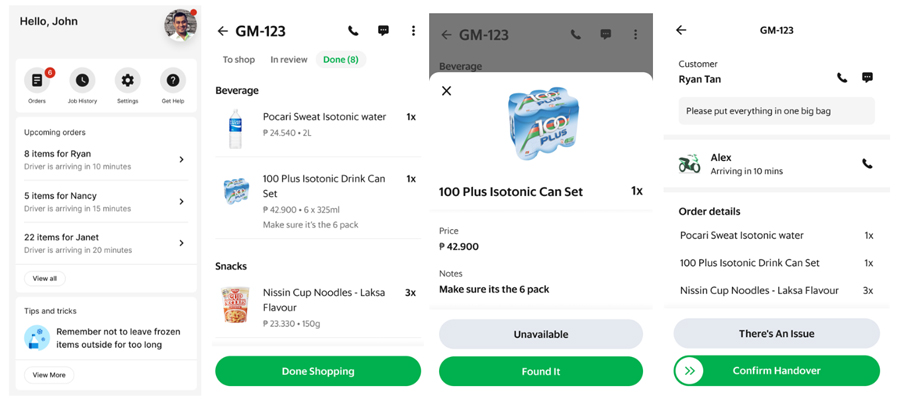The image showcases four distinct screens from the same mobile phone interface, indicating various functionalities of a delivery management app. The user is logged in, as evidenced by the "Hello John" greeting accompanied by John’s profile picture with a notification dot. 

### First Screen:
- **User Greeting:** "Hello John" 
- **Profile:** User’s photo with a notification dot
- **Upcoming Orders:**
  - **Ryan:** 8 items, driver arriving in 10 minutes (clickable for details)
  - **Nancy:** 5 items, driver arriving in 15 minutes (clickable for details)
  - **Janet:** 22 items, driver arriving in 20 minutes (clickable for details)
- **Banner:** Tips and tricks section advice, “Remember not to leave frozen items outside for too long.”

### Second Screen:
- **Section Title:** 'GM 123'
- **Beverage Listings:**
  - Popcorn
  - Sweat Isotonic Water (comment about drinking water from the tap)
  - 100 Plus Isotonic Drink (six-pack reminder)
  - Instant noodles labeled Neeson cup noodles, Alaska flavor (three units listed)

### Third Screen:
- **Section Continuation:** From ‘GM 123’
- **Product Details:**
  - 100 Plus Isotonic Can Set, priced at 42.9 units (unavailable)
  - Green button labeled "Found It" despite the unavailability

### Fourth Screen:
- **Customer Details:** Ryan Tan
- **Order Instructions:** "Please put everything in one big bag."
- **Order Arrival:** Alex arriving in 10 minutes
- **Order Summary:** Order details available upon clicking
- **Observation:** Repeated mentions of isotonic water and a general preference for it by customers.

The app provides a detailed dashboard for monitoring and managing multiple delivery orders, complete with viewing options and specific customer requests.